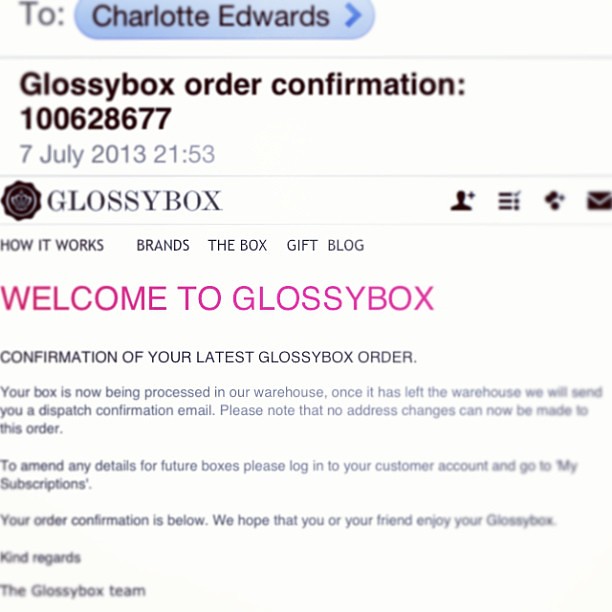This image is a detailed screenshot of an email from Glossybox to Charlotte Edwards, providing an order confirmation for her latest Glossybox purchase. The email, dated July 7, 2013, at 21:53 hours, features the order confirmation number 100-628-677. At the top, "To Charlotte Edwards" is prominently displayed, followed by "Glossybox Order Confirmation" and the date and time of the order. The header of the email highlights the Glossybox logo, adorned with a crown, and the text "Glossybox" positioned next to a navigation menu that includes "How It Works," "Brands," "The Box," "Gift," and "Blog," all aligned to the left. The welcoming statement "Welcome to Glossybox" is emphasized in bright pink letters. The email body confirms that Charlotte's box is being processed at the warehouse and mentions that a dispatch confirmation email will follow once the box has left the warehouse. The email explicitly states that no address changes can be made to the current order but provides instructions to update details for future orders through the consumer account by navigating to "My Subscriptions." Closing the email, Glossybox extends warm regards, expressing hope that Charlotte and her friend will enjoy their Glossybox. Several small icons, including a silhouette of a man with a plus sign, a menu, another icon, and an envelope, are visible but slightly out of focus at the top right of the screenshot.